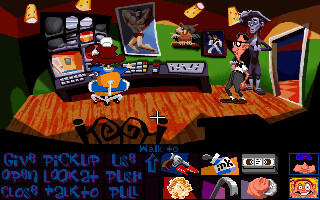The image depicts a pixelated, cartoonish scene straight out of a video game. The setting is a room with walls painted in green and orange hues. In the room, an individual is seated in an orange chair at a computer desk, which appears to be a control station with multiple screens, some active and some dormant. Above the desk, a poster featuring a muscular man in a red Speedo catches the eye. To the right, a door opens to reveal a nerdy man with glasses, a bowtie, and short hair entering the room. Behind this man stands a zombie-like statue of a pirate, adorned with a hat and featuring bulging eyes, adding an eerie touch. The room has a wooden floor, and the scene is overlaid with a classic gaming interface. The interface includes text options such as "give," "pick up," "use," "open," "look at," "push," "close," "talk to," "pull," and "walk to," along with icons representing items like ink, a gun, flames, and a crowbar.